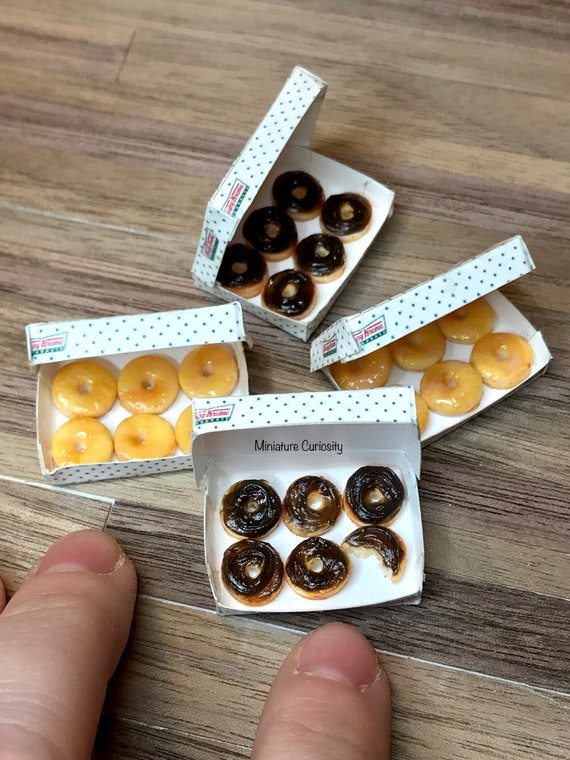The image portrays four meticulously crafted miniature boxes of Krispy Kreme donuts, positioned on a rustic wooden table with a visible natural stain that highlights its imperfections. Each rectangular box, adorned with the iconic Krispy Kreme logo in red text and green embellishments, features a white exterior dotted with green polka dots. Inside, the boxes are split between two with six chocolate-covered donuts and two with six glazed donuts, arranged in two rows of three. One of the chocolate donuts in the closest box has a conspicuous bite taken out of it, demonstrating its realistic appearance. Adjacent to the boxes are two giant fingers that serve as a scale reference, emphasizing the tiny size of these highly detailed replicas. Adding to the whimsical charm, a caption in playful font reads, "Miniature Curiosity," alluding to the handmade nature of these convincing donut miniatures.